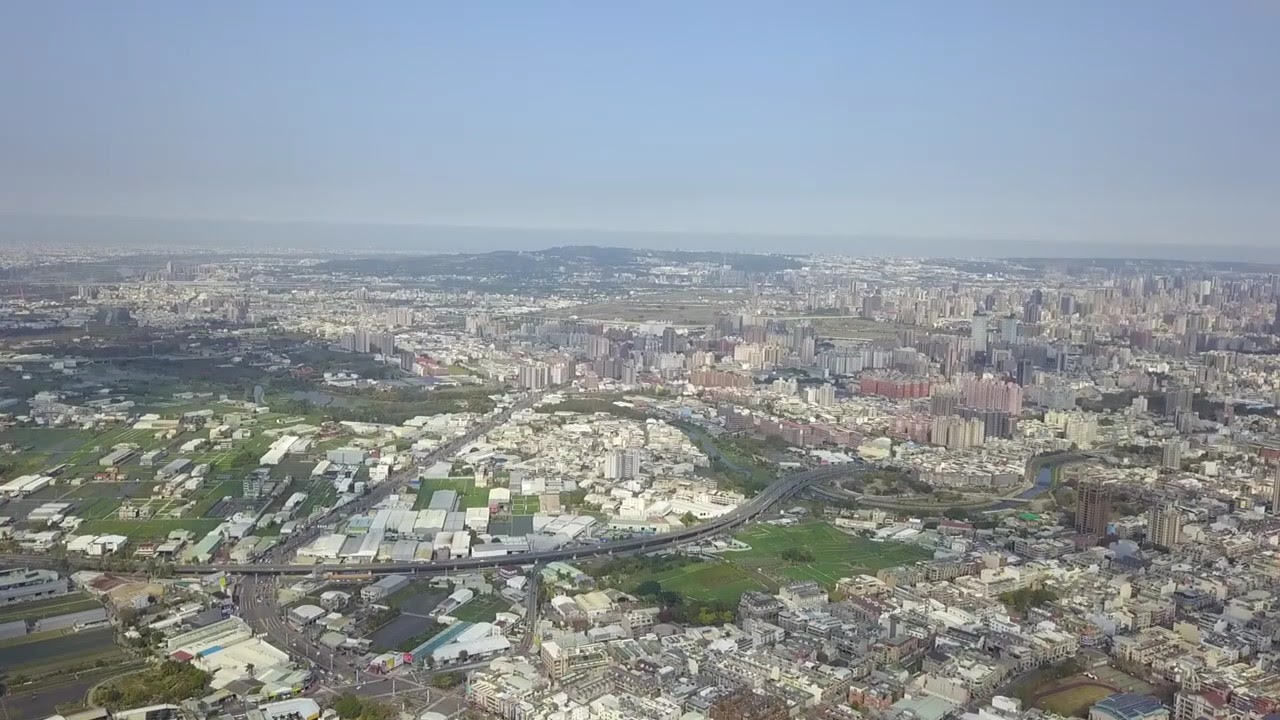This is a clear and detailed aerial photograph of a sprawling metropolis, showcasing a vibrant cityscape beneath a pristine blue sky. The lower two-thirds of the image are densely packed with hundreds of light-colored buildings, creating a mosaic of red, brown, green, black, and white structures. Interspersed among these buildings are occasional patches of greenery, particularly noticeable in the lower third center of the image. Within the lower-left quadrant, a road slices through the urban landscape, with miniature cars just discernible. 

The horizon line, occupying the upper third of the image, reveals a slight elevation, hinting at low hills or a gently hilly terrain in the distance. The sunlight, possibly during early morning or evening, casts nuanced shadows across the city, adding depth to the scene without revealing the source of light. This horizontally oriented, overhead shot captures both low-rise houses and tall high-rise buildings, altogether painting a comprehensive and dynamic portrait of the city's expanse and its varied architecture.